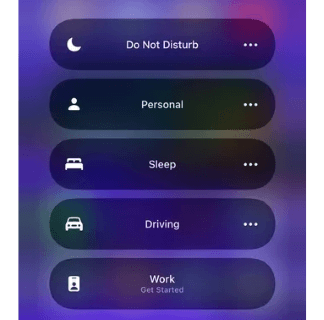The image depicts a focus management application with a hazy, purple background. The user interface features five selectable options, each represented by oval buttons. 

1. **Moon Icon**: 
   - Left: Moon emoji
   - Center: "Do Not Disturb" in white text
   - Right: Three white dots

2. **Person Icon**:
   - Left: Gender-neutral person emoji
   - Center: "Personal" in white text
   - Right: Three white dots

3. **Bed Icon**:
   - Left: Bed emoji
   - Center: "Sleep" in white text
   - Right: Three white dots

4. **Car Icon**:
   - Left: Car emoji
   - Center: "Driving" in white text
   - Right: Three white dots

5. **Badge Icon**:
   - Left: Badge emoji
   - Center: "Work" in white text
   - Below: "Get Started" directive in white text

Each option is enclosed in an oval-shaped button, enhancing the clarity and usability of the app.